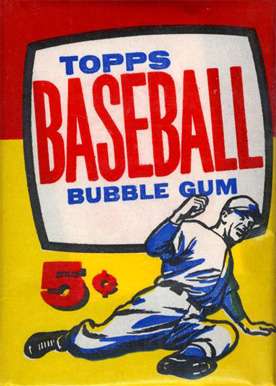This is an old-fashioned packaging design for Topps Baseball Bubblegum, reminiscent of a nostalgic era. The package features a vibrant color scheme with the top one-third painted red and the bottom two-thirds yellow. Dominating the design is a large white rectangle with a black border, spanning three-quarters of the package. Inside this rectangle, the Topps logo is prominently displayed in smaller blue all-capital letters, with "BASEBALL" written in large red capitals beneath it. Below that, the word "bubblegum" appears in smaller blue letters, all in the same font style as the Topps logo.

To the right, a red five-cent price mark stands out. The focal point is a vintage cartoon depiction of a baseball player sliding into a base. He's equipped in a traditional black-and-white baseball uniform, accented with blue on his shirt, pants, and cap. He appears to be mid-slide, with one hand touching the ground and the other arm raised, suggesting an action-packed moment. The player's position, with both legs extended and one arm in the air, vividly captures the dynamics of the game, all while reinforcing the packet's nostalgic charm.